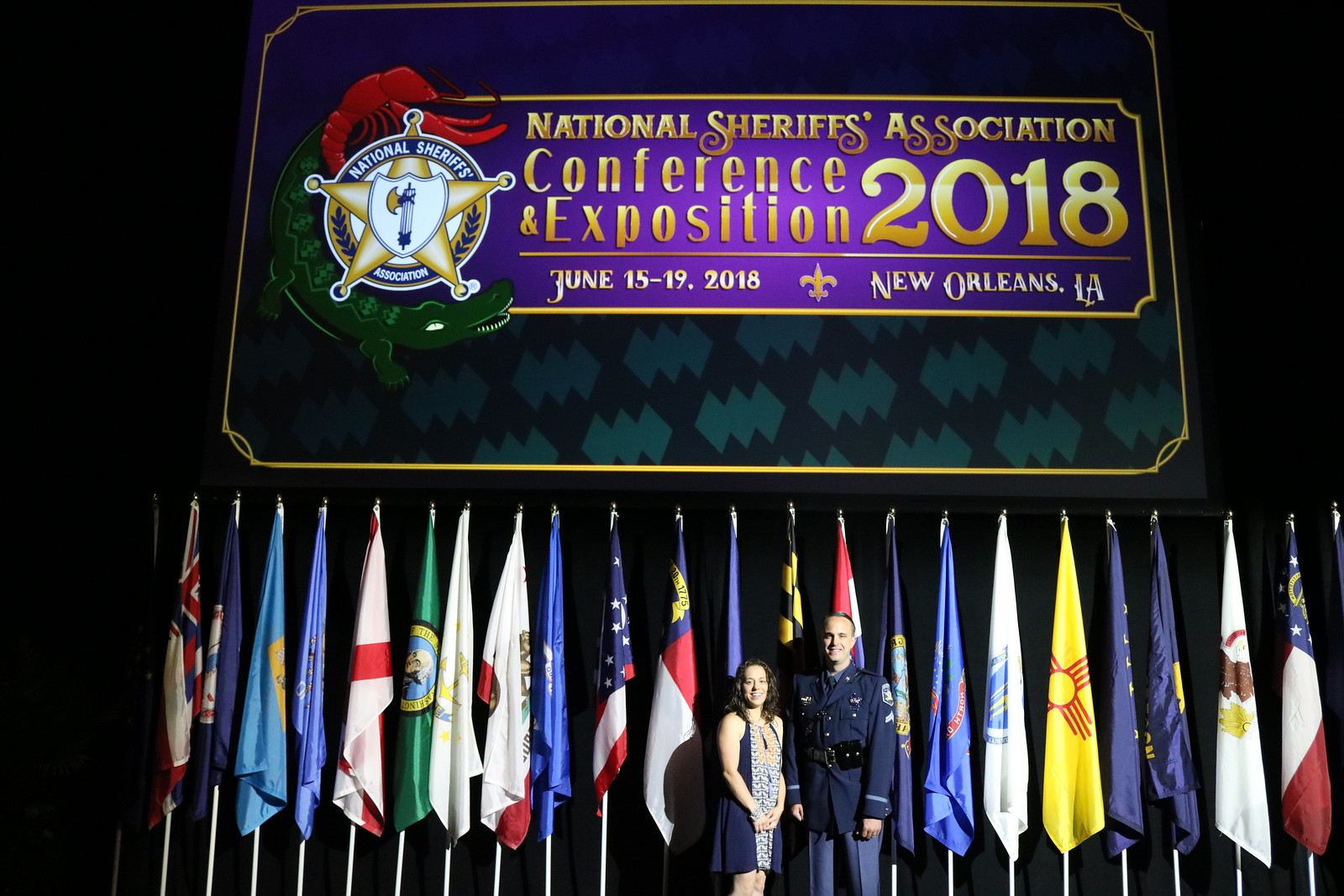In the image, two people are standing on a stage at the National Sheriffs' Association Conference and Exposition 2018, held from June 15-19 in New Orleans, Louisiana. The man appears to be a police officer or sheriff, identifiable by his uniform, while the woman next to him, who is shorter, wears a short, sleeveless, blue dress. They are both smiling for the photo. Behind them, a backdrop features numerous flags, likely state flags, arrayed against a black curtain. Above them, a large screen displays the event information in big, bold, gold lettering on a purple background, accompanied by a sheriff's badge logo that includes a gold-plated star with 'National Sheriff's Association,' encircled by an alligator and possibly a lobster motif. Additionally, a fleur-de-lis symbol is placed between the date and the location on the screen.